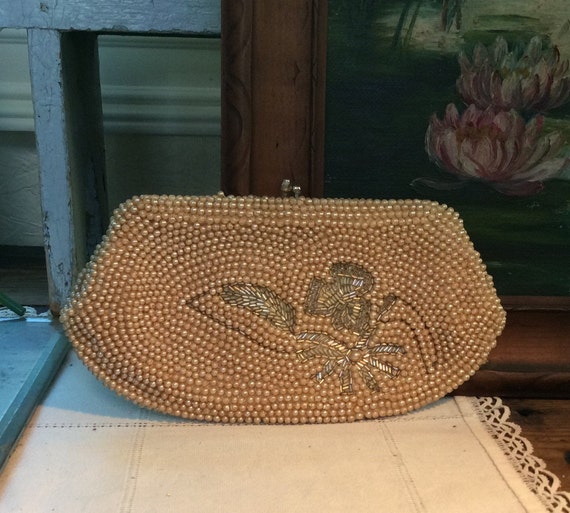The photograph captures a central focus on an aged, beaded clutch purse that exudes a vintage charm, reminiscent of the 1940s or 50s. The purse, primarily a tan or light brown color, features a delicate design in silver that resembles flowers and leaves. It’s adorned with a clasp at the top and shows signs of wear and fraying at the edges, enhancing its antique appeal. The purse rests on a cream-colored doily with lace trim, which sits atop a dark wooden tabletop. Behind the purse, there’s a framed picture, possibly depicting flowers, contributing to the nostalgic ambiance. The setting appears to be an older room with visible chair railing against the wall and a light source casting subtle shadows on the purse. The composition of the photograph highlights the purse as the main subject within a room decorated with vintage elements.